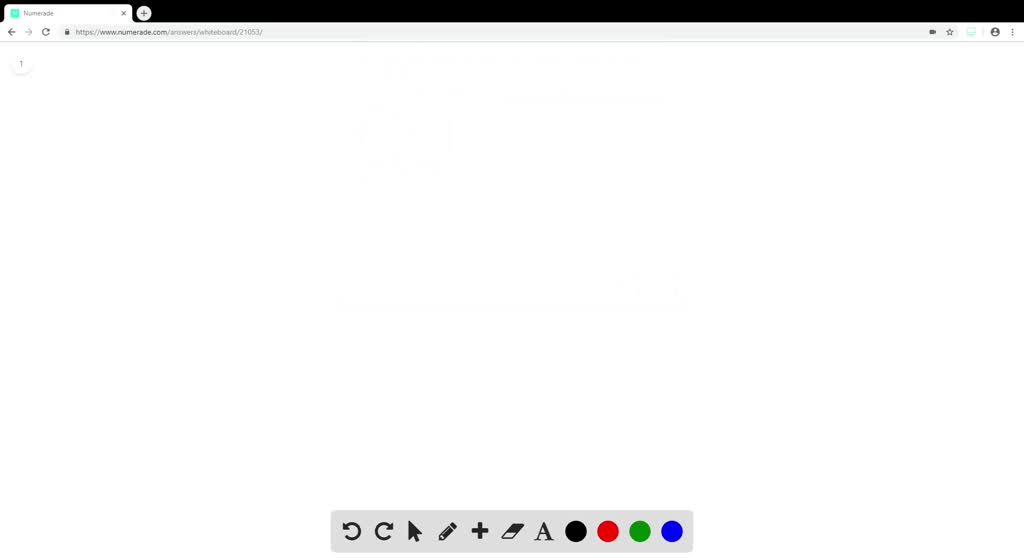This image showcases a screenshot featuring a narrow black header at the top. Below the header, on the left side, there is a small white tab open, which reads "Numerade" in slightly small font. Adjacent to this tab is a small green box. Directly below the tab is the address bar that displays the URL: "https://www.numerade.com/answers/whiteboard/21053." The majority of the image consists of a blank white background. At the bottom center of this white background, there is a small gray box containing options to choose a pencil and four circular color selections: black, red, green, and blue.